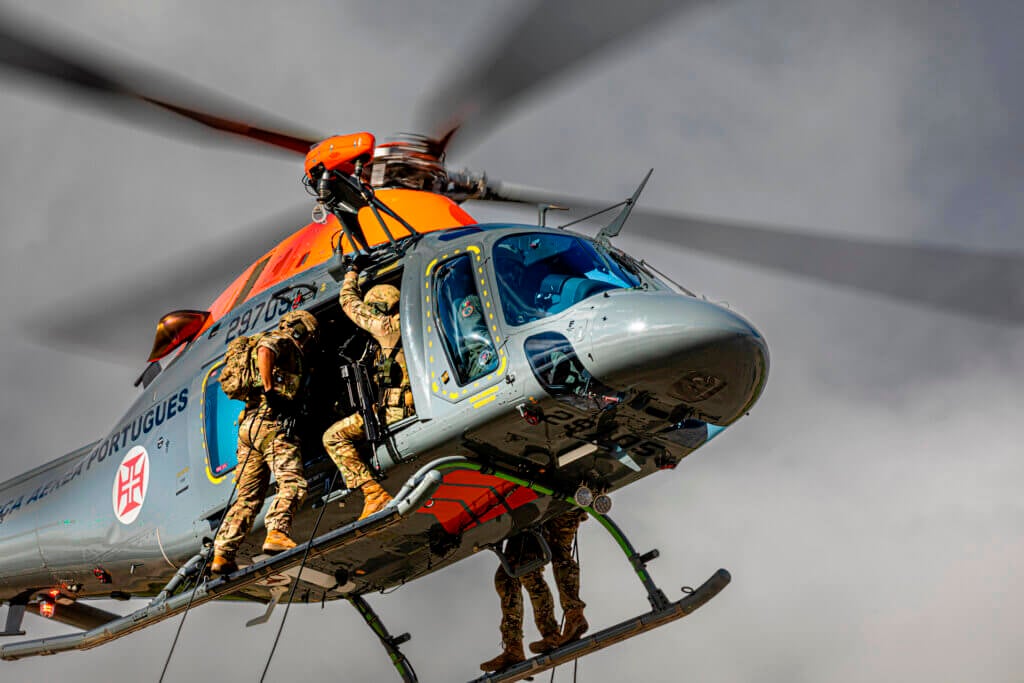In the image, a large dark grey helicopter hovers in the air against a light grey, cloud-filled sky. The helicopter features a distinct orange section atop its rotor hub, with the spinning propeller blades visibly blurred due to their high speed. Four individuals in brown and camouflage print suits, each equipped with matching helmets and orange-brown boots, are seen emerging from both sides of the helicopter. Two are poised on the left side doors, while the other two are on the right, standing on the ledge outside. They appear to be engaged in a rescue operation, evidenced by zip lines attached to their suits. On the side of the helicopter, the word "Portuguese" is clearly visible along with the number 29705, and a small emblem with a red design resembling a cross.